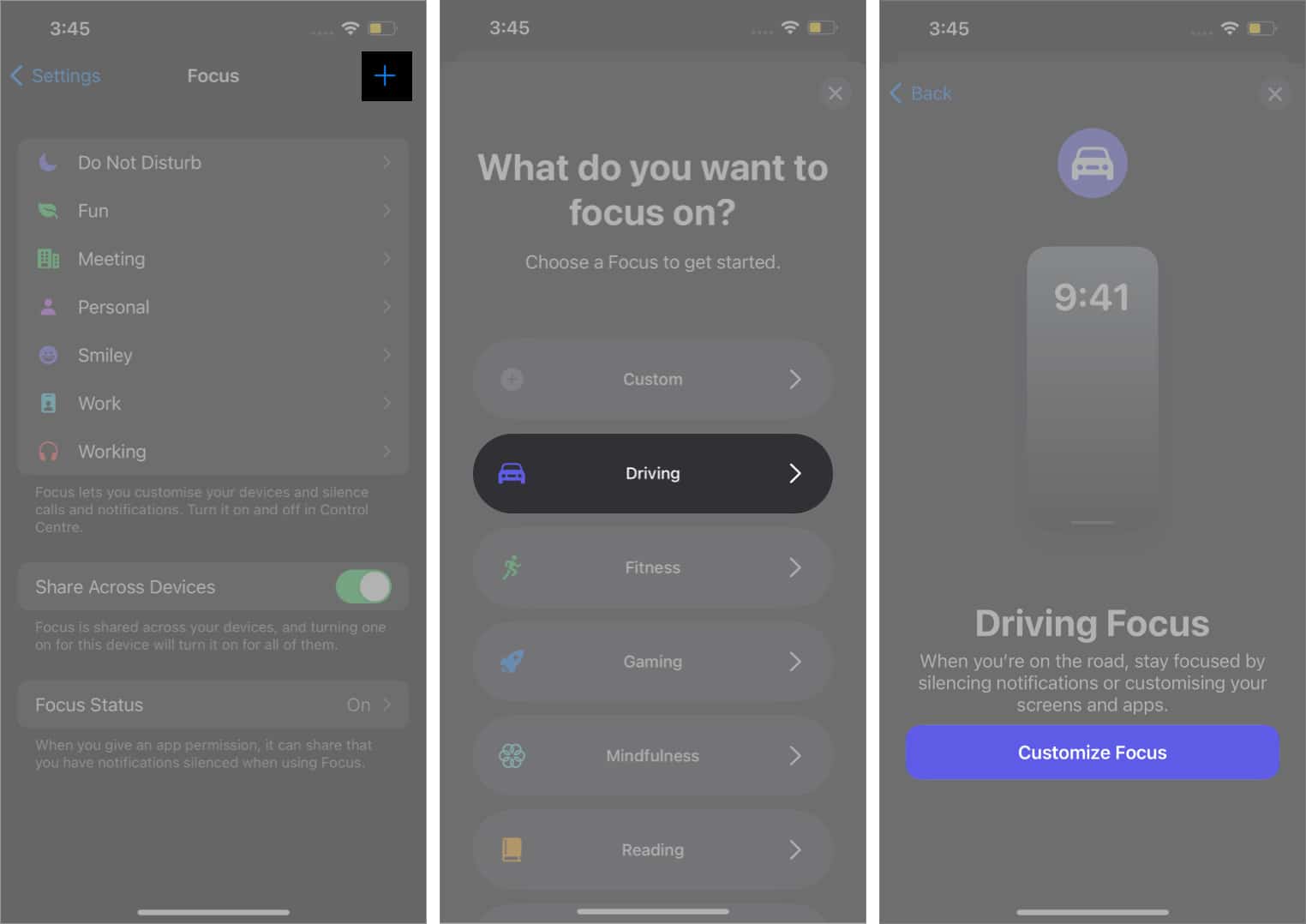In this composite image, consisting of three aligned smartphone screenshots, each bordered by a narrow white line, the background color is a uniform medium gray, creating a cohesive visual theme. 

Starting with the center screenshot, the time displayed at the top is 3:45 PM, depicted in a gray font. The header prompt reads, "What do you want to focus on?" followed by the instruction, "Choose a focus to start." Below this, a series of rectangular buttons with rounded corners are displayed as options. The top option is labeled "Custom," followed by "Driving," which is highlighted in black with white text, indicating it is selected. The remaining options listed are "Fitness," "Gaming," "Mindfulness," and "Reading."

The screenshot on the right features a small lavender circular icon at the top with a simplistic drawing of the back of a car in white. The time shown is 9:41, centered against the same gray backdrop. At the bottom, the headline "Driving Focus" is presented, accompanied by the text, "When you're on the road, stay focused by silencing notifications or customizing your screens and apps." A prominent blue rectangular button at the bottom, labeled "Customize Focus" in white text, provides an action prompt for the user.